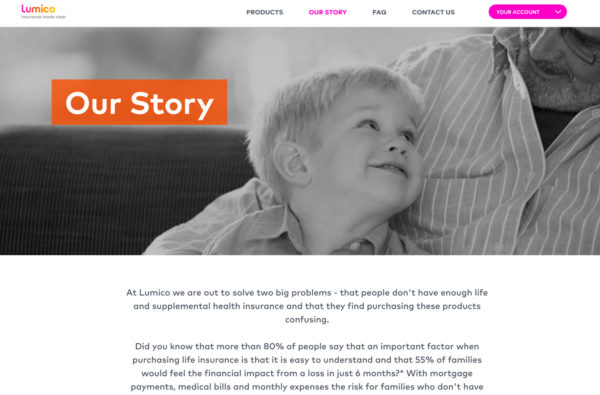This is a screenshot of a webpage from the website "Lumico." At the top left, the blurry logo reads "Lumico," with some indistinguishable text below it. The navigation bar contains four tabs: "Products," "Our Story" (highlighted in pink), "FAQ," and "Contact Us." On the top right, there is a prominent pink button labeled "Your Account."

The main content of the page features an image at the top depicting a little boy looking up at an older man, likely his grandfather or father, who has gray hair and black rectangular-framed glasses. Overlaying the top left corner of the image is the text "Our Story" in white, set against an orange rectangle. Below the image, a paragraph explains Lumico's mission: "At Lumico, we are out to solve two big problems: that people don’t have enough life and supplemental health insurance, and that they find purchasing these products confusing."